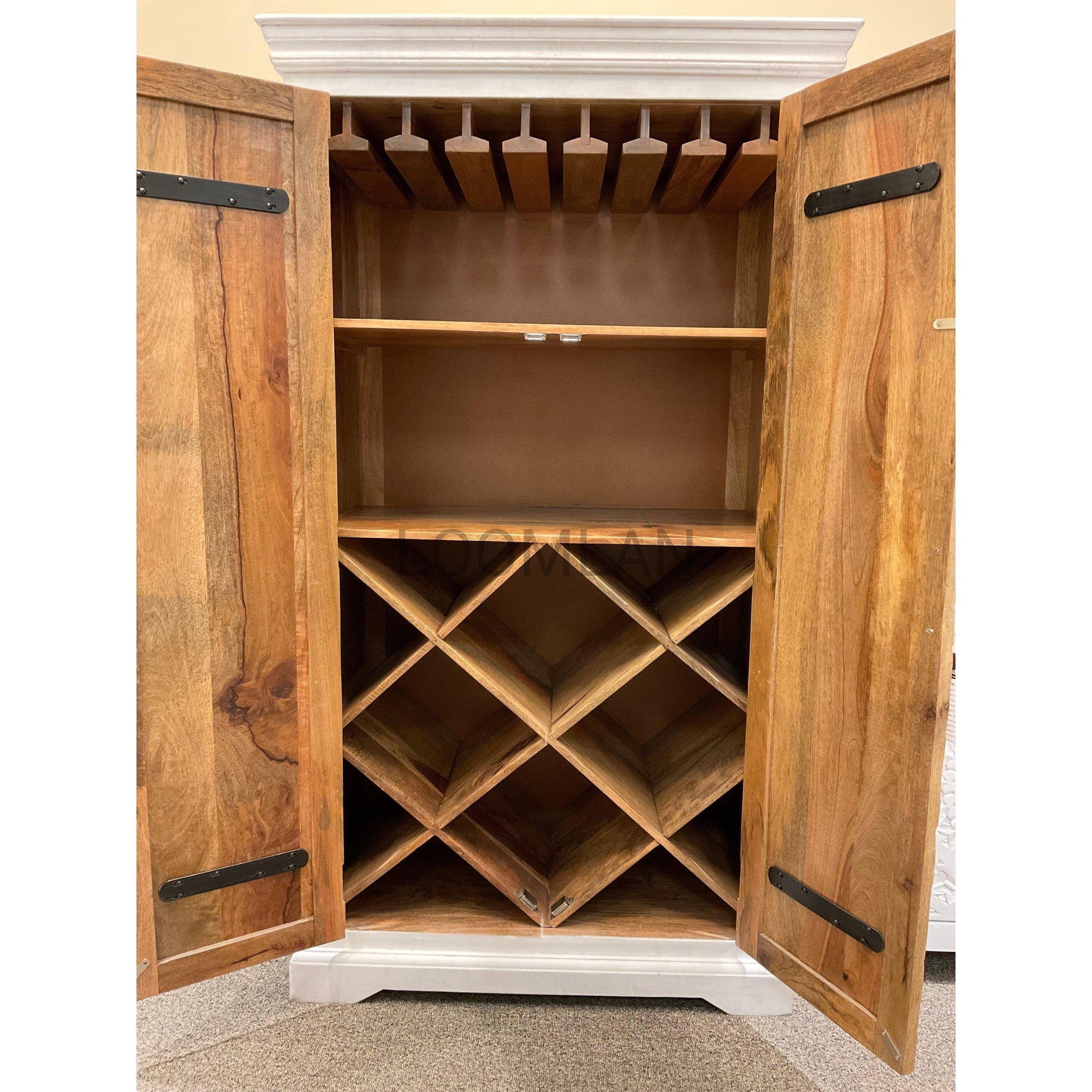This image displays a wooden wine storage cabinet with its two doors fully open to the left and right. The cabinet, primarily a light brown color, features white crown molding at both the top and bottom. The inside of each door has a black metal band running horizontally at the upper and lower thirds. At the top of the cabinet, there are racks designed to slide stemmed wine glasses for storage. Below these racks are two shelves, which could be used for standing bottles or other items. The bottom section of the cabinet features intersecting wooden pieces forming eight diamond-shaped compartments, ideal for laying wine bottles on their sides. The entire cabinet rests on a firm tan-colored floor.